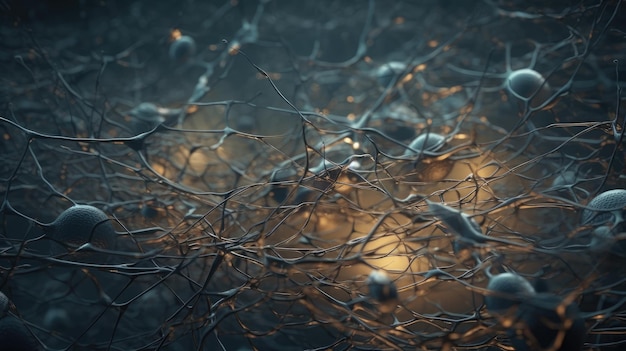This is a fascinating nature photograph dominated by a tangled network of slender, spidery branches or tendrils in a grayish-tan hue. The branches are adorned with bulbous pods or shells, which might be seed pods or animal eggs, adding an element of mystery. The overall tone of the image is dark, but a bright, yellowish light emanates from the center, creating a glowing effect that spreads throughout the photograph. The branches, appearing almost fragile and delicate, interweave in a complex, web-like pattern illuminated from below, suggesting a visual similarity to neural networks or a coral skeleton. The light brings out occasional sparkles in the middle, enhancing the photograph's intriguing and captivating nature.